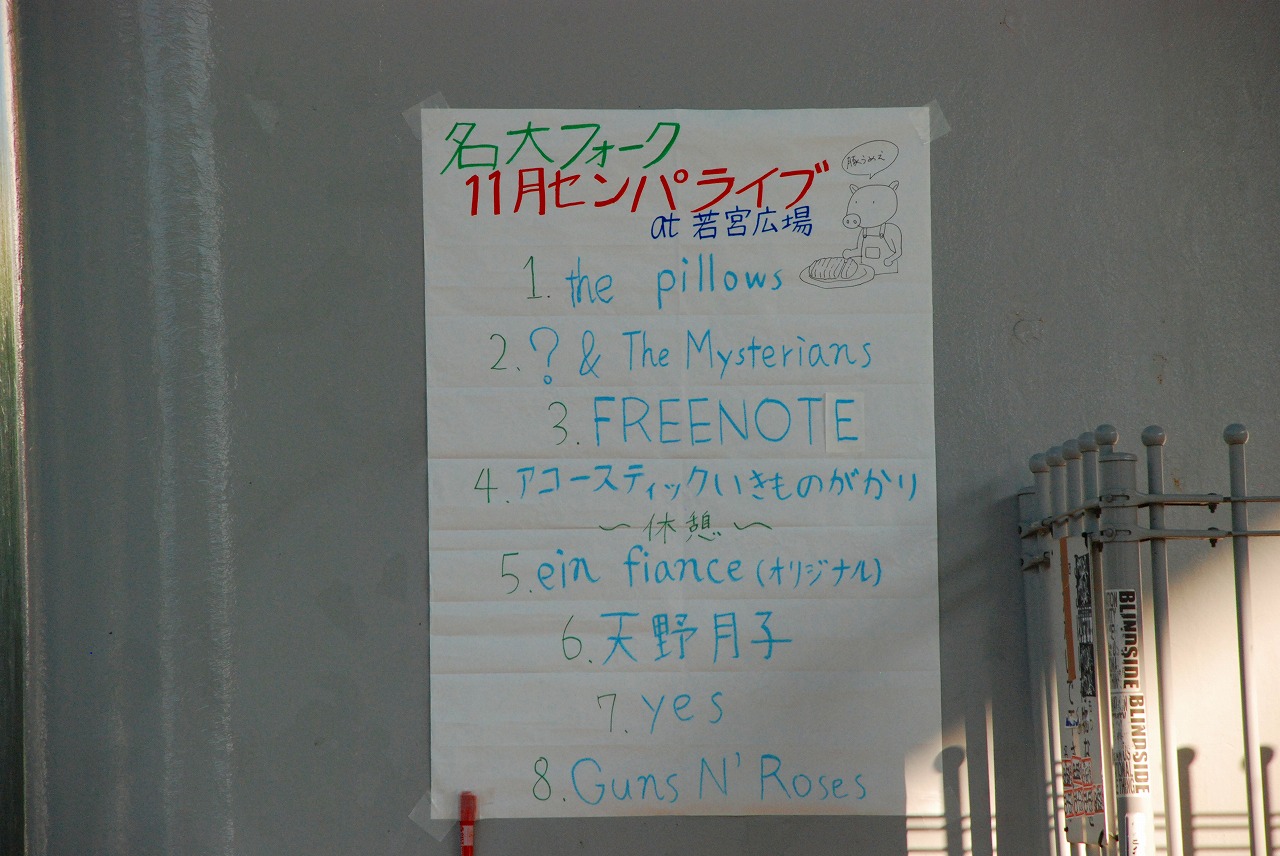The photo depicts a white poster on a grayish wall alongside a somewhat rusted and sticker-covered white metal gate, possibly in a city sidewalk setting. The poster, showing folds as if it had been unrolled before being taped up, features a striking combination of handwritten green, red, and blue text at the top in what appears to be Asian characters, potentially Thai or Japanese. Centered on the poster is a black-and-white drawing of a pig in overalls, humorously depicted as a chef preparing a plate of ham. Below this illustration is a numbered list from one to eight, which includes names resembling bands: 1. The Pillows (a known anime music contributor), 2. Question Mark & the Mysterians, 3. Freenote, 4 and 6. Entries written in Asian characters, 5. EIN Finance, 7. Yes, and 8. Guns N' Roses. The precise purpose of the list remains ambiguous without further context, adding to the overall enigmatic nature of the poster.